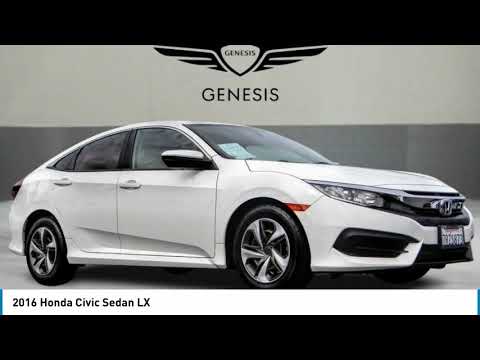The image is a slightly wider-than-tall rectangle, showcasing a sleek, white 2016 Honda Civic Sedan LX, positioned prominently in the center and facing towards the right. The car exudes a modern and sporty design with a shiny, new appearance, complete with black tires and distinctive silver hubcaps featuring fang-shaped spokes. A California license plate is visible on the front, along with a sticker on the windshield. The background is a gradient of gray, darker at the bottom and lighter above the car, creating a minimalist stage-like setting that tightly frames the vehicle. 

At the top and bottom of the image, thick black bands bookend the car, occupying about one-fourth of the total vertical height. Above the car, a light gray stripe houses the Genesis logo, which features a rounded, heart-like triangle crowned with the word "Genesis" and extending black wings. Just below this emblem, "GENESIS" is printed in large capital letters. At the bottom of the image, a white band with the inscription "2016 Honda Civic Sedan LX" in plain black font runs below the car, capturing essential model details. The composition and tight framing of the shot emphasize the car's sleek lines and modern aesthetics, making it the focal point against the unassuming backdrop.